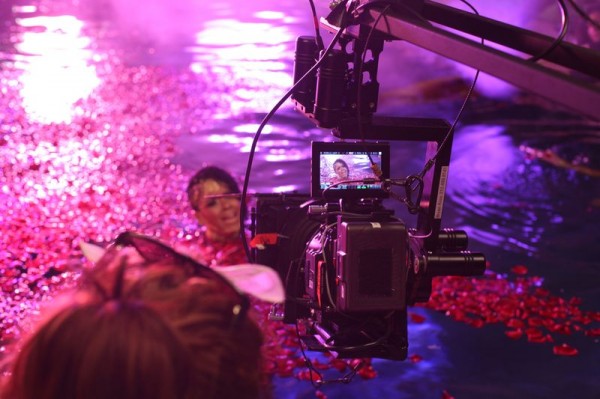In this vibrant and artistic scene, a black female artist is being filmed while partially submerged in a river-like pool at night, which is part of the making of a music video or commercial. The pool is artistically adorned with pink petals or glittery elements that float and scatter around her, lending a magical and colorful ambiance to the setting. The water around her shimmers with soft blues, purples, and pinks, as lights reflect off the surface, creating an enchanting atmosphere. She is emerging from the water, holding or wearing a maroon-colored blanket or dress that adds to the mystique of the image. She gazes directly into the camera with a subtle smile. A camera operator, possibly female, is visible holding a camera and boom, capturing this mesmerizing scene through a viewfinder that displays the woman's serene and captivating presence amidst the vivid and dreamy backdrop.